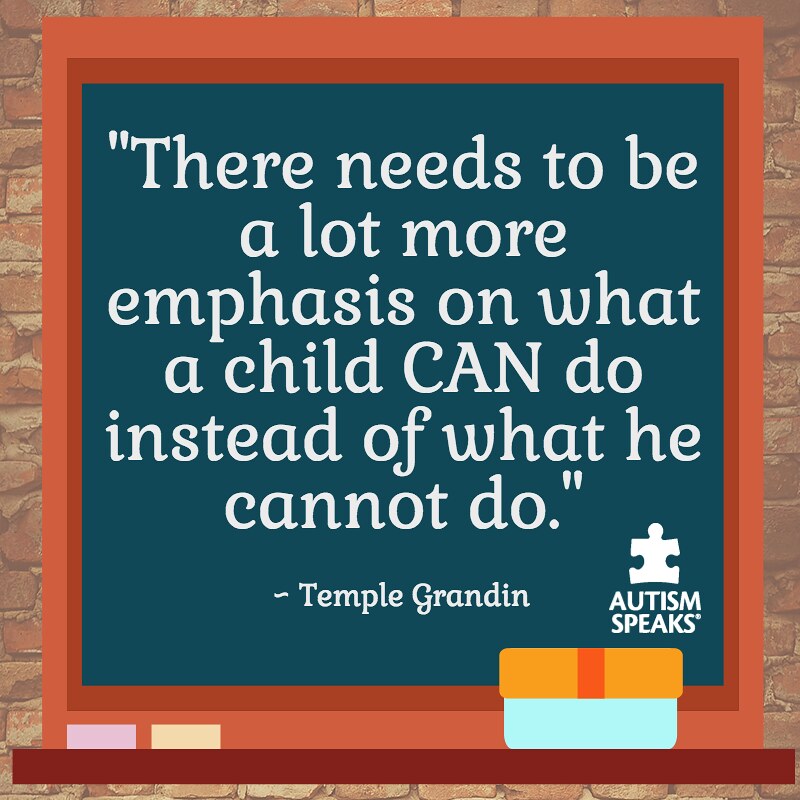The image is a digitally generated piece featuring a motivational quote prominently displayed on a sign mounted against a brick wall, suggesting an outdoor setting in broad daylight. The sign, situated centrally in the image, has a detailed, multi-layered frame. The outermost border of the frame is dark red, followed by an inner orange border. Additional elements adorn the frame, including small purple and yellow rectangles at the bottom left corner and a design resembling a blue box with yellow and orange accents at the bottom right.

The center of the sign has a dark blue background, resembling a blackboard, and bears the following quote in white text, with "can" emphasized in capital letters: "There needs to be a lot more emphasis on what a child can do instead of what he cannot do," attributed to Temple Grandin. Below the quote, a white puzzle piece logo appears, with the words "Autism Speaks" beneath it, indicating the organization's involvement. The image's vibrant color palette includes brown, orange, off-green, white, gray, yellow, light blue, and purple, contributing to its eye-catching appearance, likely designed to convey a motivational message for sharing on social media or as part of an advertisement.